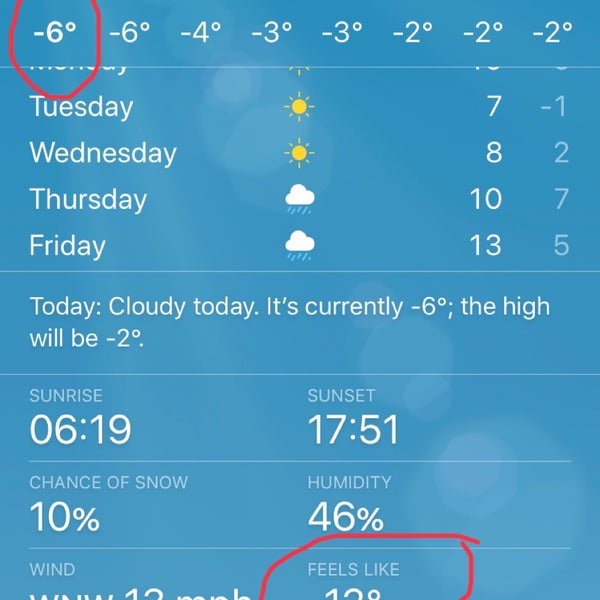This image shows a highly detailed weather website interface, predominately colored in blue with white text and numbers. At the forefront, there are multiple temperature readings displayed in negative figures, such as -6, -6, -4, -6, -3, -3, -2, -2, and 2. The first -6 is distinctly circled in red marker. Below the temperatures, weekdays are listed, though Monday is partially cut off. Each day's weather forecast includes a mix of sunshine and rain indicators. 

Specifically, Tuesday through Friday are forecasted with high temperatures of 7°C, 8°C, 10°C, and 13°C, respectively. The low temperatures for Tuesday span from -1°C to 5°C. A section marked "Today" describes current conditions as cloudy, with a current temperature of -6°C and a high of -2°C. Further details mention a 10% chance of snow, 46% humidity, and wind speeds at 12 miles per hour. Sunrise is noted at 6:19 AM and sunset at 9:51 PM. The "feels like" temperature is partially visible and suggested to be around 12 degrees based on the visible top of the one and curvature of the two, also highlighted with a red marker.